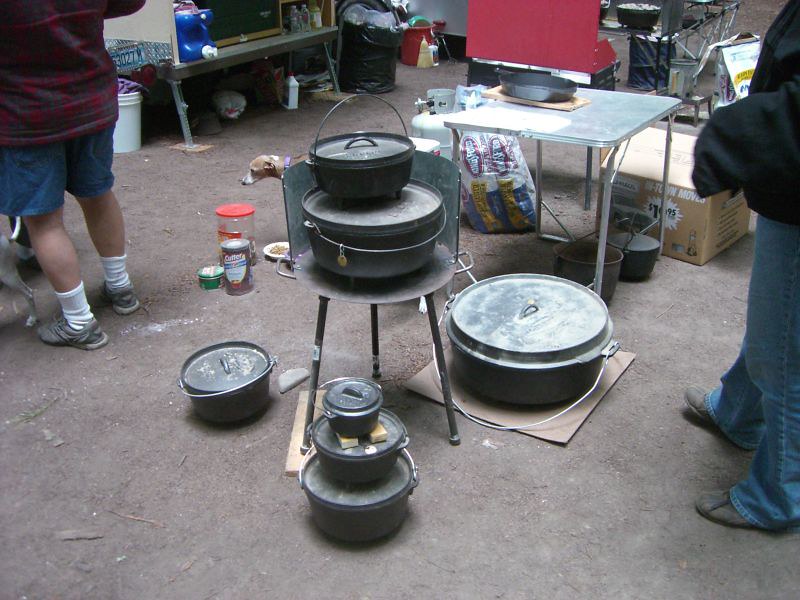The photo depicts an outdoor scene, taken during a somewhat cloudy yet bright day, set on a concrete ground. Dominating the foreground, there are multiple cooking pots and pans of various sizes, many with lids. A particularly large cast iron pot that appears suitable for camping stands out, alongside six smaller pots. These pots and pans are partially stacked, with some arranged on a chair and others positioned directly on the ground. 

There’s a juxtaposition of household and grilling items, including a folding table and another table behind it laden with cooking essentials. Beneath the tables and scattered around are two large bags of charcoal, several seasoning containers, and a box. Additionally, the scene includes a silver table, a laundry detergent dispenser, and in the background, a sizable grill designed for outdoor cooking.

To the right of the image, a person is visible from the waist down, dressed in jeans and gray shoes, suggesting they may be wearing a hoodie or long-sleeve top. On the left, another person appears from the mid-back down, clad in jean shorts, gray tennis shoes, white socks, and a plaid shirt. A curious dog peeks out from behind one of the tables, adding a touch of liveliness to the scene. All together, the array of items and the figures hint at preparations underway for a substantial cookout.